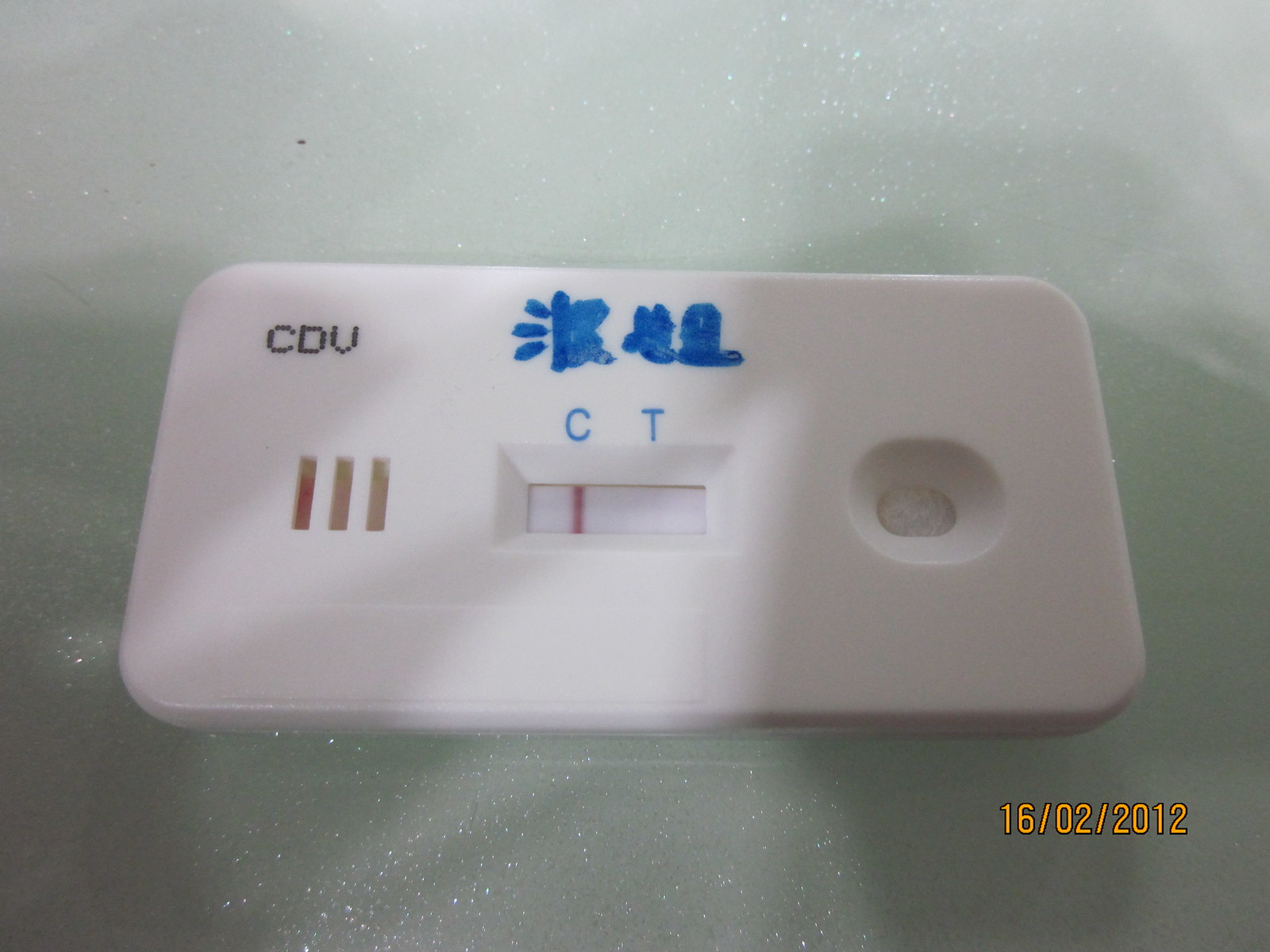The image depicts a medical testing kit resembling a COVID-19 test, although it predates the pandemic by several years. The device, white with a smooth plastic surface, sits on an almost white, glass-like surface. In the top left corner, it has "CDV" inscribed in black text and features hand-written Asian characters in blue marker, the meaning of which is unclear. 

Central to the device are the letters "C" and "T" in blue, spaced apart. A red line is visible beneath the "C," which likely indicates a test result. On the left side, the device has three small indentations whose purpose is unspecified. There is a small divot on the right side, probably intended for the application of a sample, such as blood or saliva.

A date, "16-02-2012," is printed in orange at the bottom right corner, indicating the European date format of February 16, 2012. Given the date, it suggests that this device may be an early form of diagnostic testing, possibly used for detecting diseases like the flu that could have influenced the design of later COVID-19 test kits.